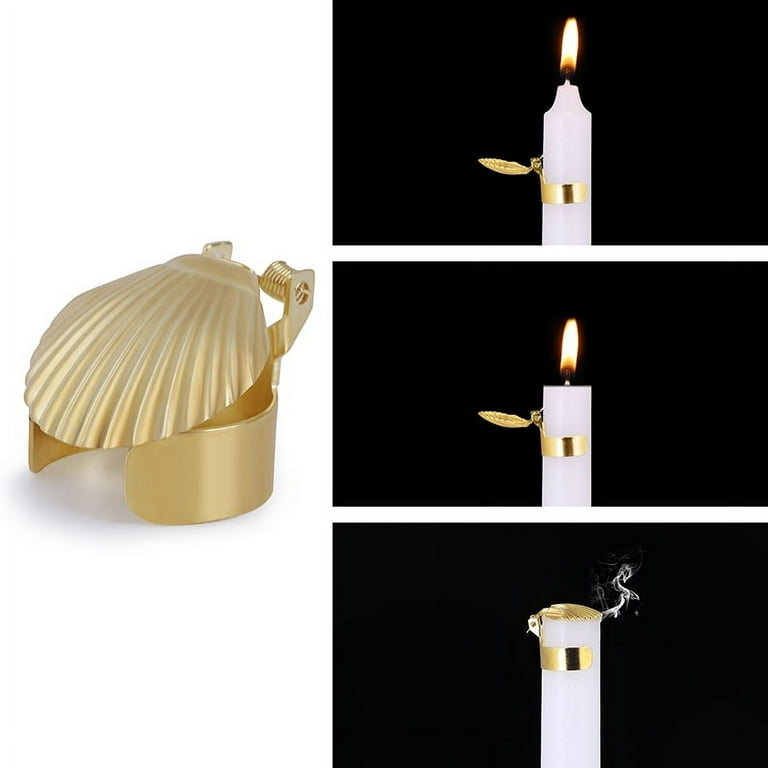The image comprises a modern set of three sequential photographs on a black background, illustrating the functionality of a gold candle stopper shaped like a scallop seashell. On the left side of the image, there's a detailed close-up of the golden scallop seashell stopper, which can open and close over the candle. In the first photograph on the right, the white candle is newly lit, with the golden seashell stopper in an open position some distance above the flame. The second photograph shows the candle burning halfway down, with the stopper having moved closer to the flame. In the third photograph, the candle has burned down far enough for the stopper to automatically close over the extinguished flame, with a puff of smoke rising to indicate that the flame has been put out. The sequence graphically demonstrates the self-activating mechanism of the candle stopper, designed to safely extinguish the candle’s flame as it burns down.